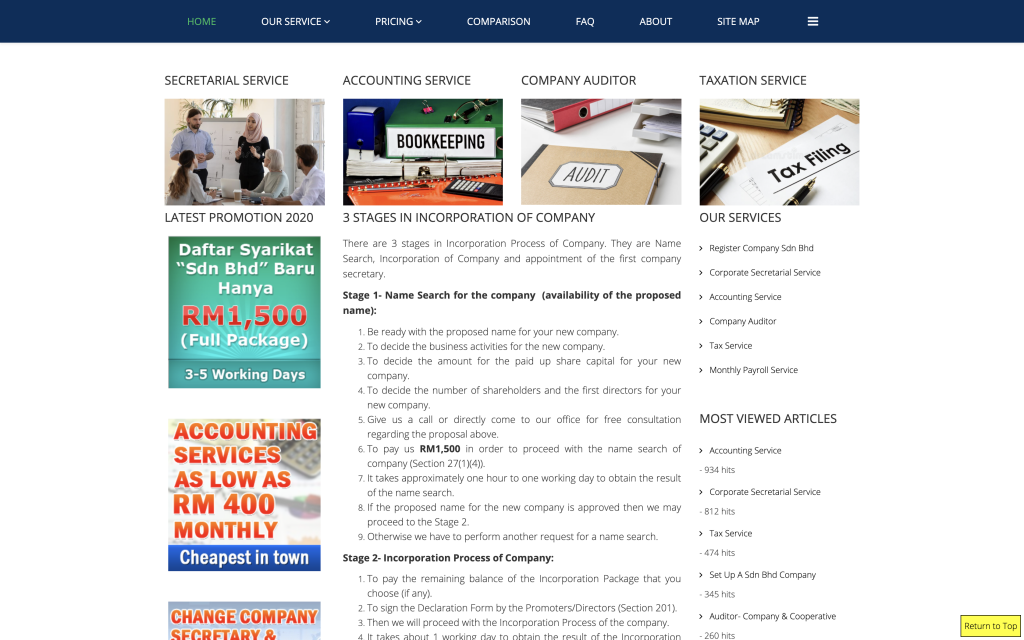A screenshot of a professional services website, though the specific name of the website is not visible in the screenshot. Positioned at the top of the page is a dark navy blue banner that includes navigational links: Home, Our Service (with a drop-down menu), Pricing (with a drop-down menu), Comparison, FAQ, About, Sitemap, and a Hamburger menu.

The website is divided into seven main sections:
1. Secretarial Service
2. Accounting Service
3. Company Auditor
4. Taxation Service

Along the right-hand side are two or three advertisements.

Each listed service is accompanied by a corresponding stock image.

Beneath the services, there is a section titled "Three Stages in Incorporation of Company" which details the stages involved in the incorporation process: Name Search, Incorporation of Company, and Appointment of the First Company Secretary.

To the right of this text, there's a sidebar labeled "Our Services," which lists several services offered by the business: Register Company, Corporate Secretarial Service, Accounting Service, Company Auditor, Tax Service, Monthly Payroll Service.

Below this, another section lists "Most Viewed Articles." At the bottom right corner of the page, there's a yellow "Return to Top" button for easy navigation back to the top of the page.